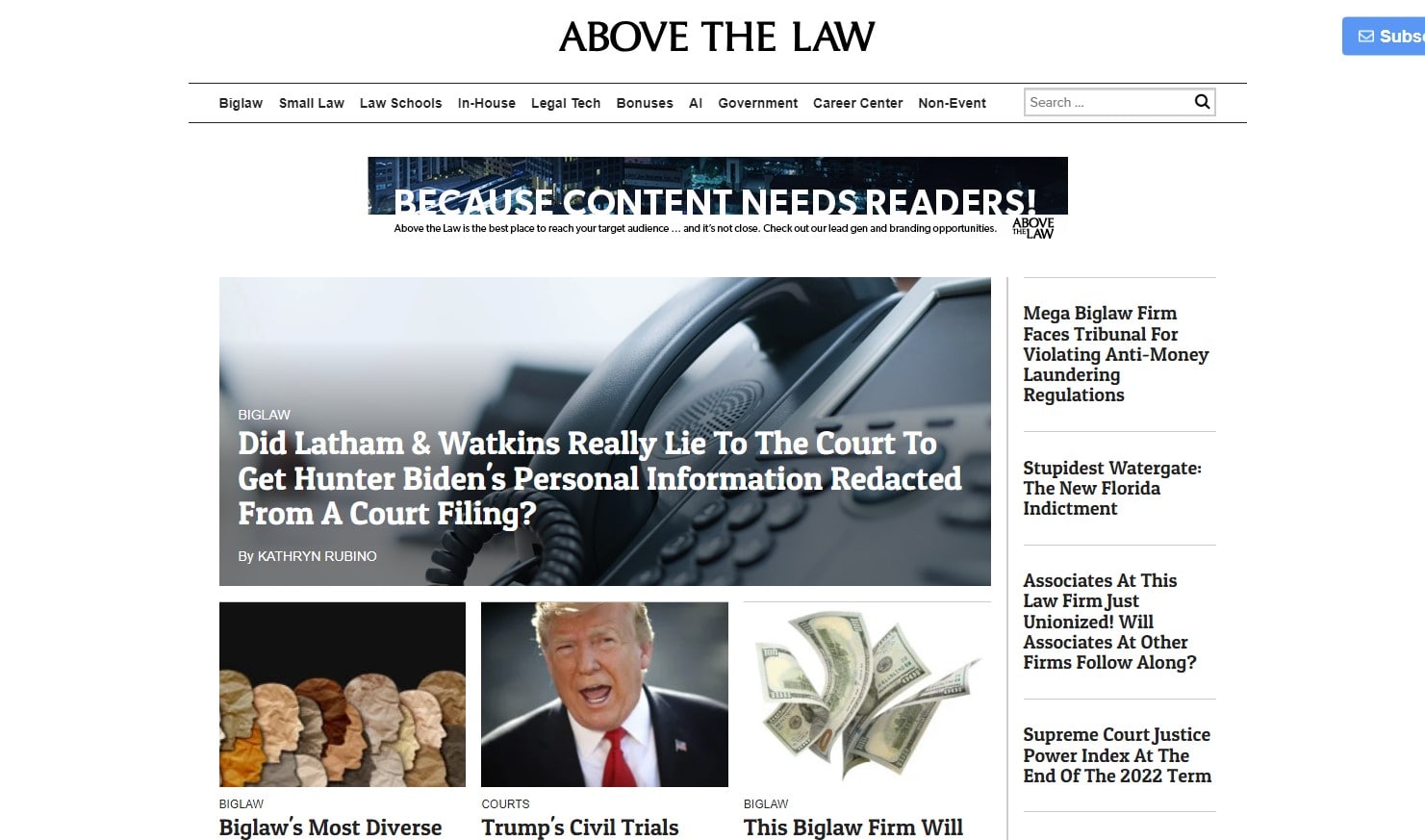In the image of the website, we see a detailed layout of a legal news platform. At the very top, the website title "Above the Law" is prominently displayed in a large black font. To the right of the title, there is a subscribe button, although part of it is obscured.

Below the header, a navigation menu lists various categories in black text, from left to right: Big Law, Small Law, Law Schools, In-House, Legal Tech, Bonuses, AI, Government, Career Center, and Non-Event. Adjacent to these categories on the right-hand side, there is a search bar.

Underneath the navigation menu, a subheading reads, "Because Content Needs Readers," followed by a black-colored sentence just below it.

On the left side of the page, we see several article headlines. The first article questions, "Did Latham and Watkins really lie to the court to get Hunter Biden's personal information redacted from a court filing?" Just below this, an article titled "Big Law is Most Diverse" is accompanied by an image showing side-view rock faces. 

Adjacent to these, we find "Trump's Civil Trials," which features a picture of Trump. To the right of this article, another entry titled "The Big Law Firm" is shown next to an image of money.

In a column to the right, four additional article titles are listed in black text:
1. "Mega Big Law Firm Faces Tribunal for Violating Anti-Money Laundering Regulations"
2. "Stupidest Watergate: The New Florida Indictment"
3. "Associates at This Law Firm Just Unionized: Will Associates at Other Firms Follow?"
4. "Supreme Court Justice Power Index at the End of the 2022 Term"

The layout and design efficiently categorize and present various legal articles and topics, aiming to engage readers with diverse and current legal content.